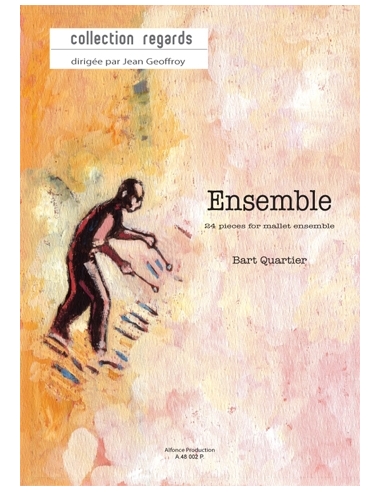The image prominently features a well-centered book cover set against a solid white background. The cover, vertical in format, is filled with artistic, collage-like elements in a palette of orange, pink, black, white, and varying shades of brown. Dominating the cover is a stylized, cartoon-like drawing of a balding man wearing glasses and dressed in light brown or reddish-toned clothing, holding mallets in each hand as he appears to play an abstract marimba.

Text elements on the cover include "Collection Regards" in a white horizontal box at the top left, followed by "Dirige Per Jeanne Girouffe Ensemble," "24 Pieces for Mallet Ensemble" in smaller print, and the name "Bart Courtier" at the bottom. The large word "Ensemble" is positioned on the middle right in black text. The artistic backdrop complements the minimalist yet detailed depiction of the man, enriching the overall visual impact of this book cover, which might easily be mistaken for an art exhibition program or a high-quality magazine.